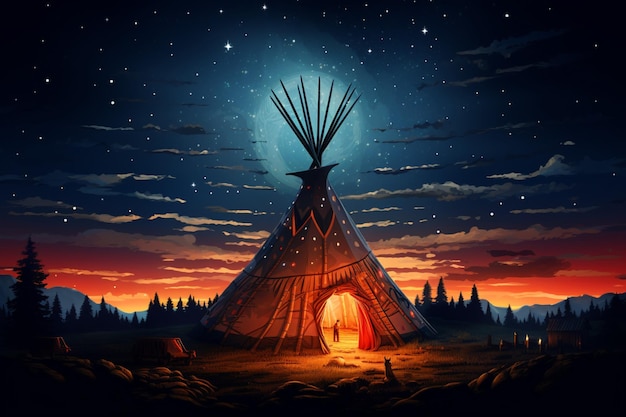The image features a vividly animated illustration of a large, highly decorated Native American tipi, seemingly AI-generated. The tipi is constructed with sticks that extend upwards and is illuminated by a warm orange light, which makes it glow brightly from the inside. The opening reveals a small, disproportionately tiny figure standing within, giving an almost fantastical element to the scene. The tipi is situated in the heart of a dense forest, surrounded by numerous tall trees and earthy ground.

The sky above is a prominent feature, blending shades of blue, red, and yellow hues that suggest a transition from sunset into night. Stars glitter across the sky, accompanied by a crescent moon and gray clouds. The overall atmosphere of the scene is magical and serene, with a sense of peaceful solitude. The presence of an animal near the tipi adds to the enchanting, almost mystical quality of the setting.